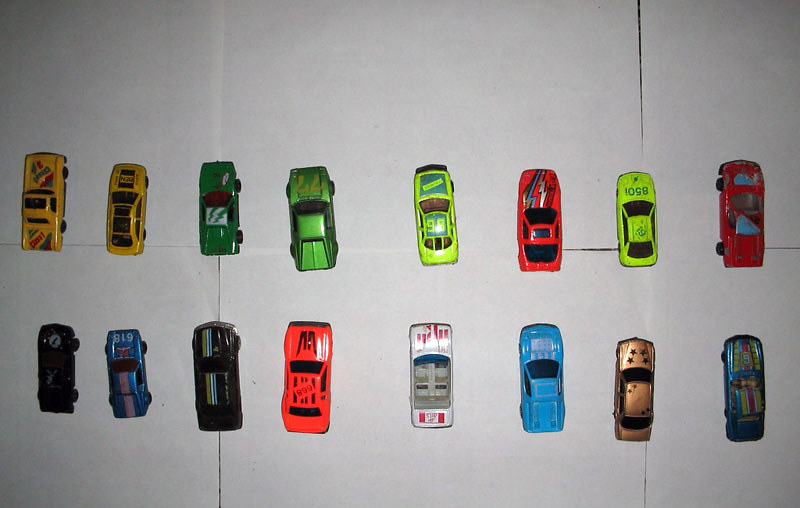The image showcases 16 matchbox or Hot Wheels-style cars, meticulously arranged in two rows of eight on a grid of white squares formed by overlapping sheets of paper. Photographed from a top-down perspective, the cars are oriented uniformly, with their fronts facing the top and rears toward the bottom of the picture. The cars, uniform in size but varying in design, boast an array of vibrant colors including shades of yellow, orange, green, red, blue, bronze, and black. Notably, the collection features a gray convertible with a red design on the front and a pickup truck, adding to the diversity. Some cars exhibit a newer sheen while others appear vintage, hinting at a rich assortment. The top row starts with two yellow cars followed by a light green, a hot pink, a green, and a red car. The lower row presents a black car, a blue one, another black car, and a red car, with a notable white convertible centrally positioned. Additionally, specific details such as the green car marked with '8501' and the yellow, blue, and red car stamped with the number '6' enhance the intricacy of the display.